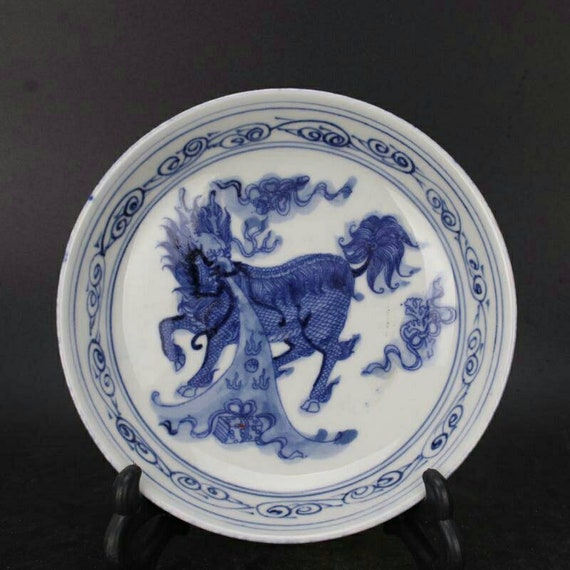This image captures a detailed, intricately designed decorative plate on a black stand, set against a dark background. The medium-sized white plate features a blue motif dominated by a central figure that resembles a fantastical horse or dragon. This creature, adorned with a flowing mane and bushy tail, seems to be emitting a fiery stream from its mouth. At the end of this flame-like stream, there appears to be a gift-wrapped package. Surrounding the central figure are interconnected blue swirls forming a border, punctuated by alternating two thin circular blue lines. Additional blue figure-eight patterns or ribbon-like designs embellish the plate's perimeter. The combination of the vibrant blue detailing against the white porcelain creates a striking visual contrast, all perfectly supported by the plate's black display stand.